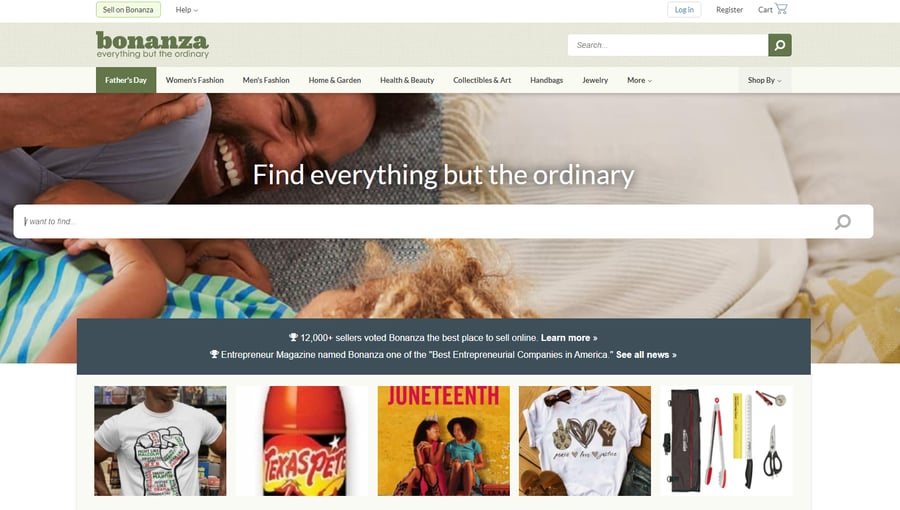The image portrays the homepage of a website belonging to the company Bonanza. The company's logo, "Bonanza," is prominently displayed in lowercase letters at the upper left corner, accompanied by the tagline "everything but the ordinary" in an olive green hue.

At the very top-left, there's a clickable tab inviting users to "Sell on Bonanza," and to its right, a drop-down menu offers help options. On the upper right-hand side, there's a series of links: a cart button to view your shopping cart, followed by "Register" and "Login."

Directly below the logo and tagline is a search bar, allowing users to find specific items. The website features a horizontal navigation menu with tabs categorized into "Father's Day" (highlighted in the same olive green), "Women's Fashion," "Men's Fashion," "Home and Garden," "Health and Beauty," "Collectibles and Art," "Handbags," "Jewelry," and a "More" drop-down menu for additional categories. On the far right is another drop-down menu labeled "Shop By."

The main section of the webpage is dedicated to "Father's Day", showcasing a themed highlight with the phrase "Find Everything But The Ordinary". Behind this text is an engaging image of a father playing with his daughter, enhancing the thematic focus. Below the search bar, the site provides further information about Bonanza, and the lower section of the screen features a selection of five random images, presumably showcasing various products or categories available on the site.